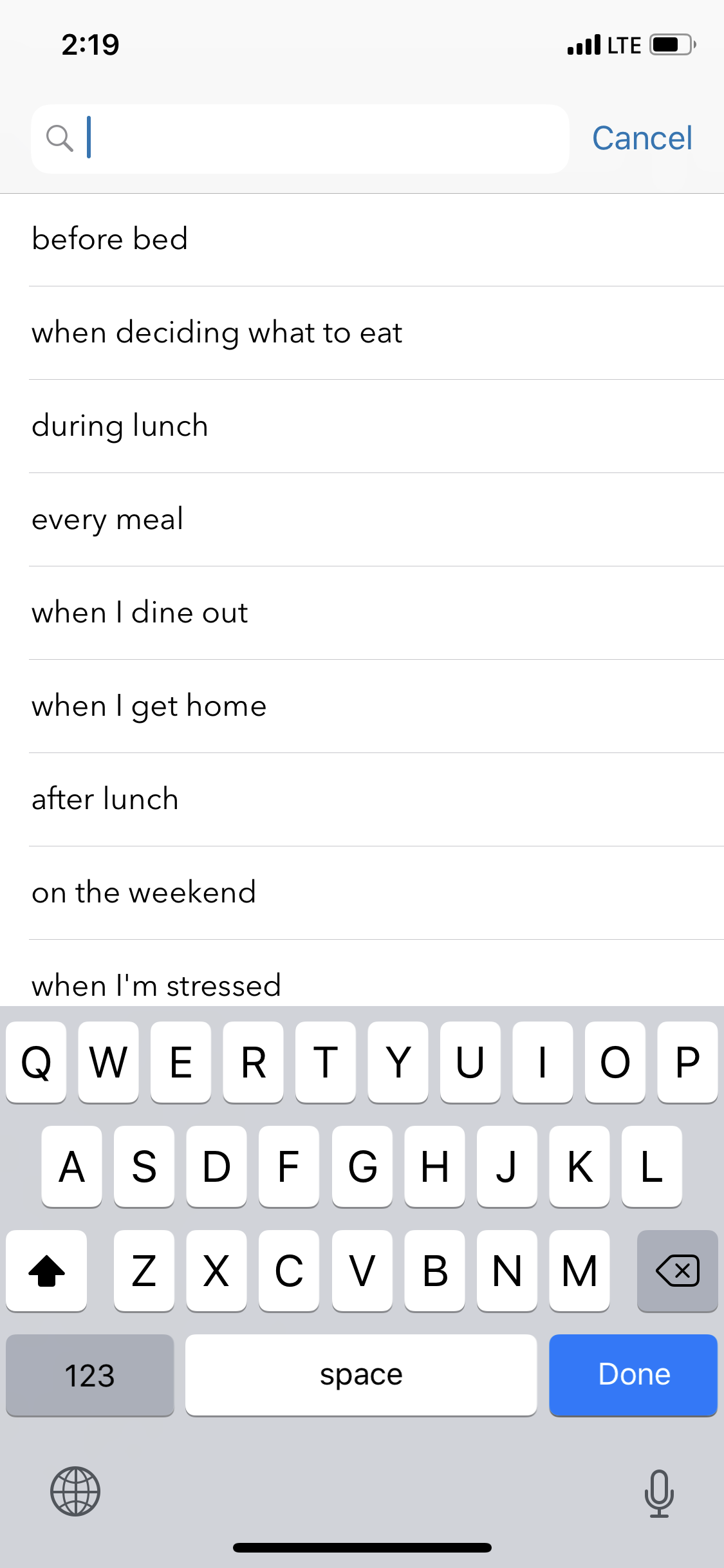This screenshot, captured at 2:19 PM on a cell phone, displays a variety of information and user interface elements. The top of the screen shows full bars of cellular service and the "LTE" indicator, alongside a battery icon that appears to be approximately 60% charged. Dominantly featured is a search bar with a blue blinking cursor, magnifying glass icon, and the word "Cancel" in blue text on the right-hand side.

Below the search bar is a list of search suggestions, each separated by horizontal dividers. The suggestions read as follows: 
- "Before bed"
- "When deciding what to eat"
- "During lunch"
- "Every meal"
- "When I dine out"
- "When I get home"
- "After lunch"
- "On the weekend"
- "When I'm stressed"

At the bottom portion of the screenshot, the standard QWERTY keyboard layout of the phone is visible, ready for text input. All elements combined provide a clear representation of a search activity in progress on a mobile device.